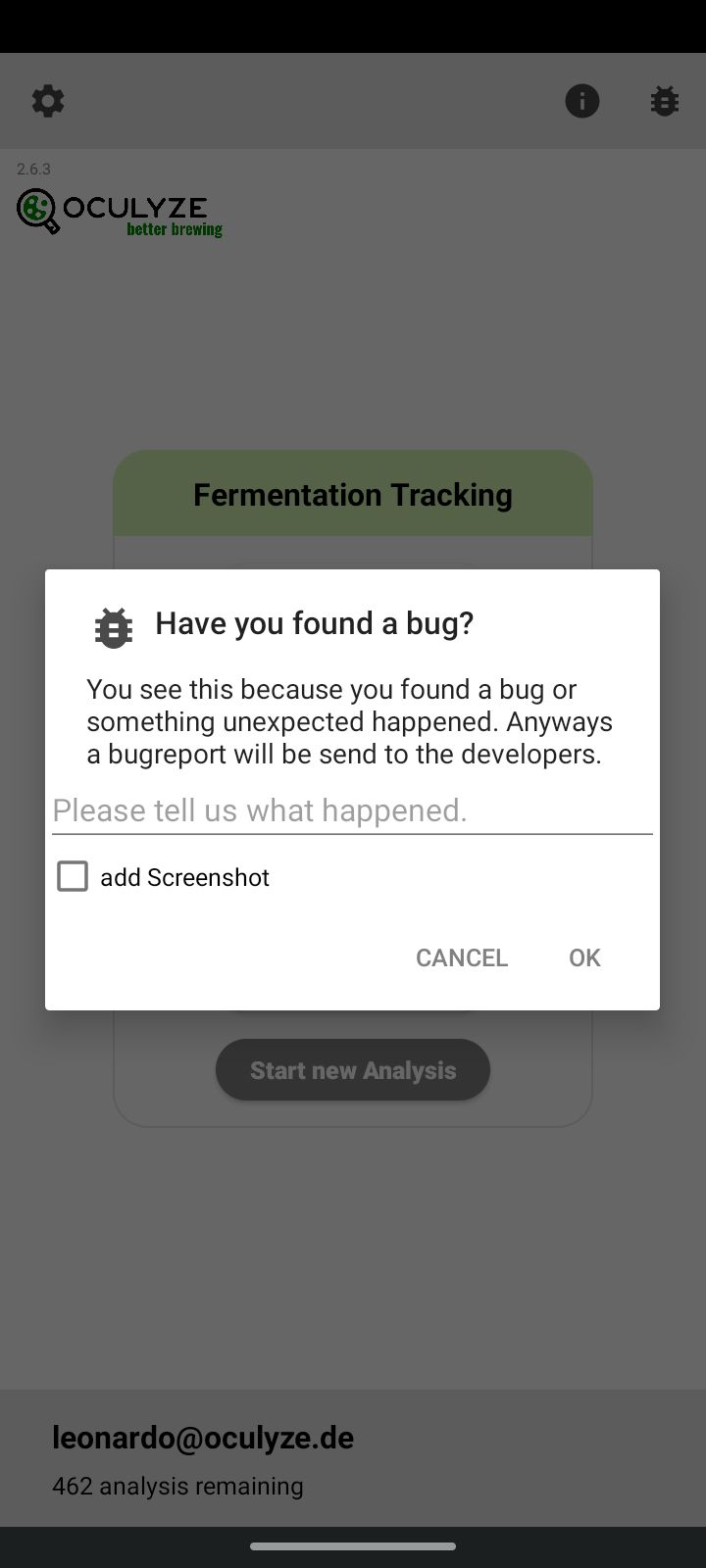**Caption:**
The image depicts a smartphone screen predominantly white in color, highlighting an interface from a company called Oculize. Central to the screen is a circular gear icon labeled "I" with the words "Oculize: Better Investing, Better Browsing" above it. The screen also features a section titled "Start New Analysis" under a logo associated with Oculize. The company's contact person, Leonardo, can be reached at Leonardo@Oculize.de.

Additionally, the screen displays a bug report window with the message: "Have you found a bug? You see this because you found a bug or something unexpected happened. A bug report will be sent to the developer. Please tell us what happened." Below this message are options to "Add screenshot," "Cancel," and "Okay." The display further includes a segment detailing 462 analyses from A-Wing.

The bottom of the screen is somewhat out of focus, leading to a condensed aspect ratio of the graphical user interface displayed on the phone.